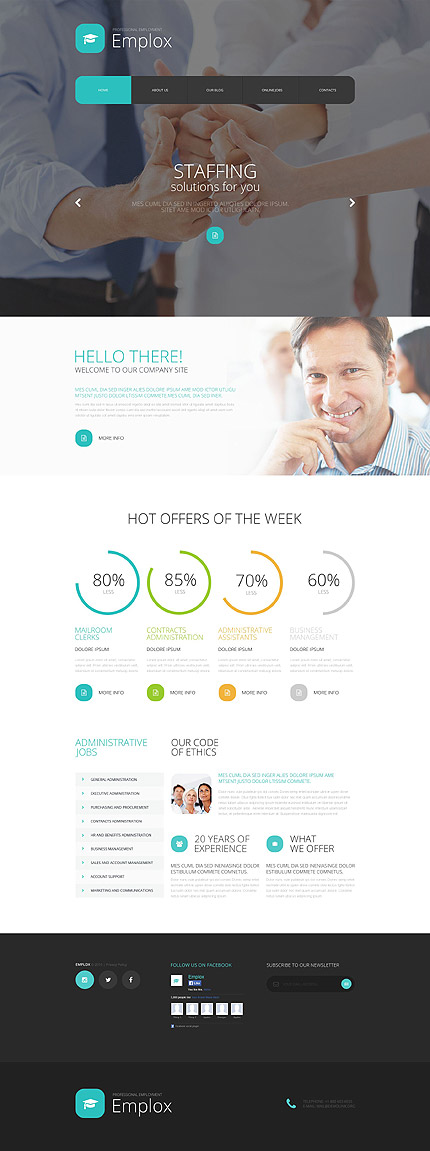**Descriptive Caption:**

The image is a detailed screenshot of a website displayed on a phone. The top third of the screen showcases a central picture of four hands, all giving thumbs up and touching at the thumbs. These hands are positioned as follows: one hand extends from the left, another from the right, and two more from the upper right, all uniformly dressed in white long-sleeved dress shirts.

Approximately an inch from the top left corner, there is a prominent blue square with white lines. To its right, the logo "EMPLOX" (spelled twice: M-PLOX, E-M-P-L-O-X) is visible in white text. Beneath this logo, there is a blue tab followed by four black tabs, each with white writing. Centrally positioned, bold white text states "STAFFING," with a subheading beneath it that reads "Solutions for you." Below this, there are two lines of text in a foreign language. Adjacent to these, a blue circle with white content is noticeable.

Further down, the right side of the screen features an image of a smiling man, finger on chin, with brown hair and a blue-and-white striped shirt, looking directly at the camera. Behind him, an African American woman and a white woman are visible. To the left of this image, in large, bold, blue, all-capital letters, the words "HELLO THERE" are displayed, followed by the black text "Welcome to our company site." Below this greeting are two lines of blue text and three lines of black text containing additional information. A blue clickable tab labeled "MORE INFO" is also present.

The section below this displays text in black against a white border, announcing "Hot offers of the week." This segment is followed by a sequence featuring a three-quarters blue circle, green circle, orange circle, and gray circle, each containing percentage figures and the word "Less" underneath them. 

Continuing down the page, the names and details of classrooms are listed, followed by a section on the left labeled "Administrative Jobs" with nine listings beneath it. An adjoining section titled "Our Code of Ethics" includes a descriptive paragraph. Further down on the left side, the text reads "20 years of experience" with another explanatory paragraph. On the right side, a section titled "What we offer" is accompanied by a corresponding paragraph. The bottom of the screenshot reveals a black bar with multiple clickable links for navigating to different parts of the website.

This comprehensive depiction provides a thorough overview of the webpage and its contents.